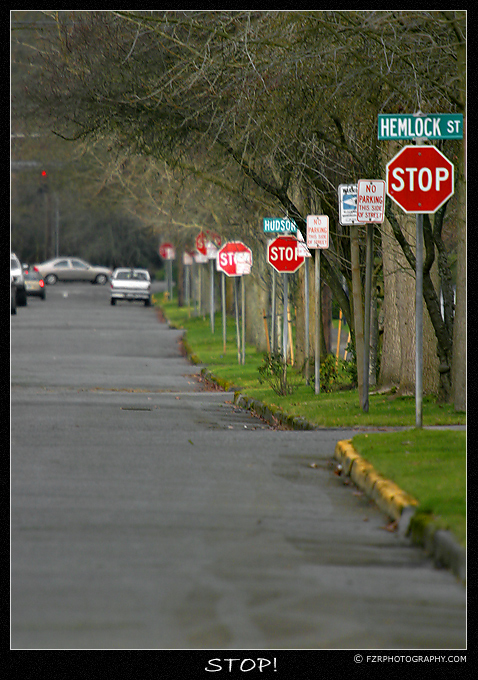The image is a poster-sized color photograph framed by a thin black border on top and sides, with a slightly thicker black border at the bottom. Dominating the poster is an almost humorous scene of a neighborhood street lined with an unusual number of stop signs. The perspective is looking down the center of this street, where at least seven stop signs are visible or partially visible in a grassy culvert area on the left, interspersed by various side streets intersecting from the right. Above the stop signs are street signs, notably "Hemlock Street" and "Hudson Street." The right side of the main street features some curbing, with occasional yellow safety paint, alongside grassy patches.

Scattered throughout the grassy strip are additional signs, including no parking signs and a warning neighborhood watch sign. In the distant background, cars can be seen, one navigating a different street and another traveling down the main street. The street surface appears somewhat bumpy, and the overall ambiance is slightly overcast, adding a gray tone to the scene.

At the bottom of the poster, in large capital letters, the word "STOP!" punctuates the message, reflecting the abundance of stop signs. In the bottom right corner, the photographer's credit appears along with a copyright notice, "fzrphotography.com." The scene is an amusing, exaggerated portrayal of urban street signage, emphasizing the sheer number of stop signs in view.